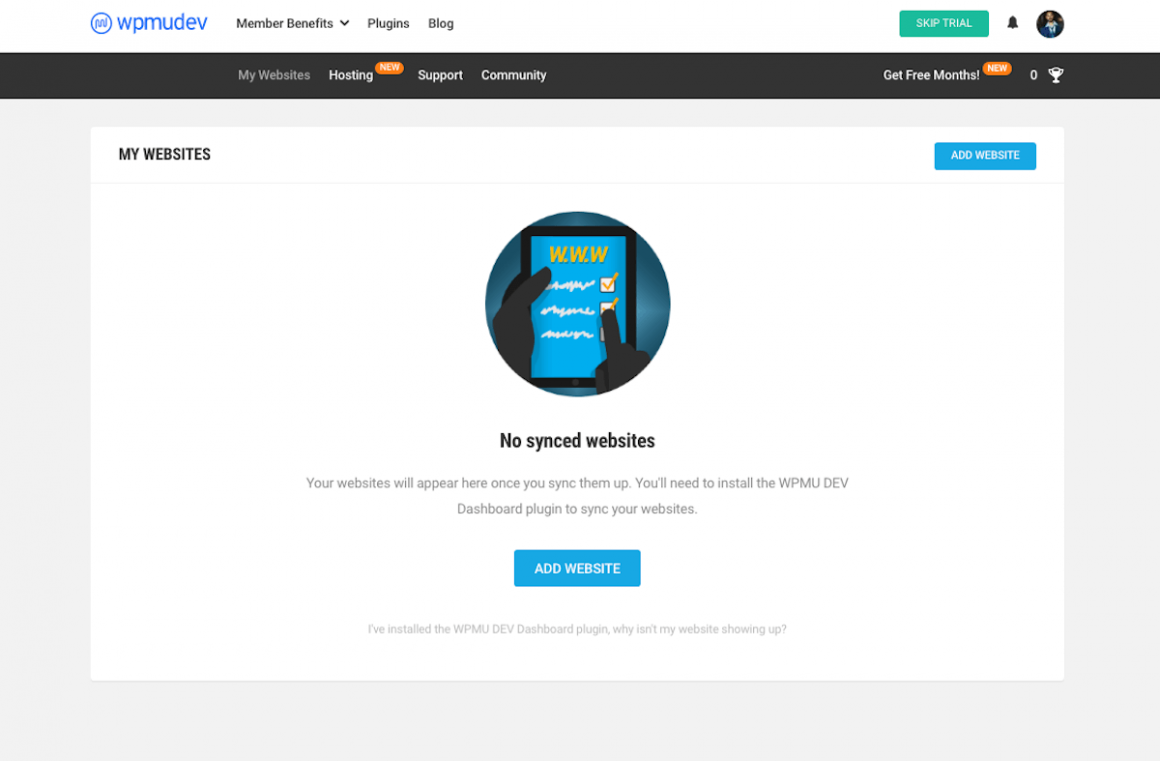### Detailed Descriptive Caption:

The image is a rectangular screenshot of a website, where the long side of the rectangle spans from left to right. At the very top, there's a layered border: a thin white strip followed by a thicker black strip, setting off the main content area of the page.

In the top left corner, the word "WPMUDEV" is displayed in blue text. Adjacent to this, in black text, are the menu options: "Member Benefits," "Plugins," and "Blog."

A green box is positioned on the left side of the screen, featuring white text that reads, "Skip Trial." Alongside this box, a notification symbol and a circular icon, representing an account (with a person's silhouette inside), are evident.

On the black border, the left side includes navigation labels: "My Websites," "Hosting," "Support," and "Community." On the right side, there’s a prompt reading "Get Free Months" next to an orange box with the word "New" highlighted, indicating a recent feature, likely related to hosting.

"My Websites" is the currently selected option. Below this, within a white content section, the heading "My Websites" is prominently displayed. A message within this section states, "No Synced Websites. Your websites will appear once you sync them up. You'll need to install the WPMUDEV dashboard plugin to sync your websites."

Toward the bottom of this section, there is a blue box with white text that reads, "Add Website." Similarly, a smaller blue box with the same label is located in the upper right-hand corner of the white section. This entire white section is enclosed by a subtle gray border, providing a clear delineation from the rest of the page.